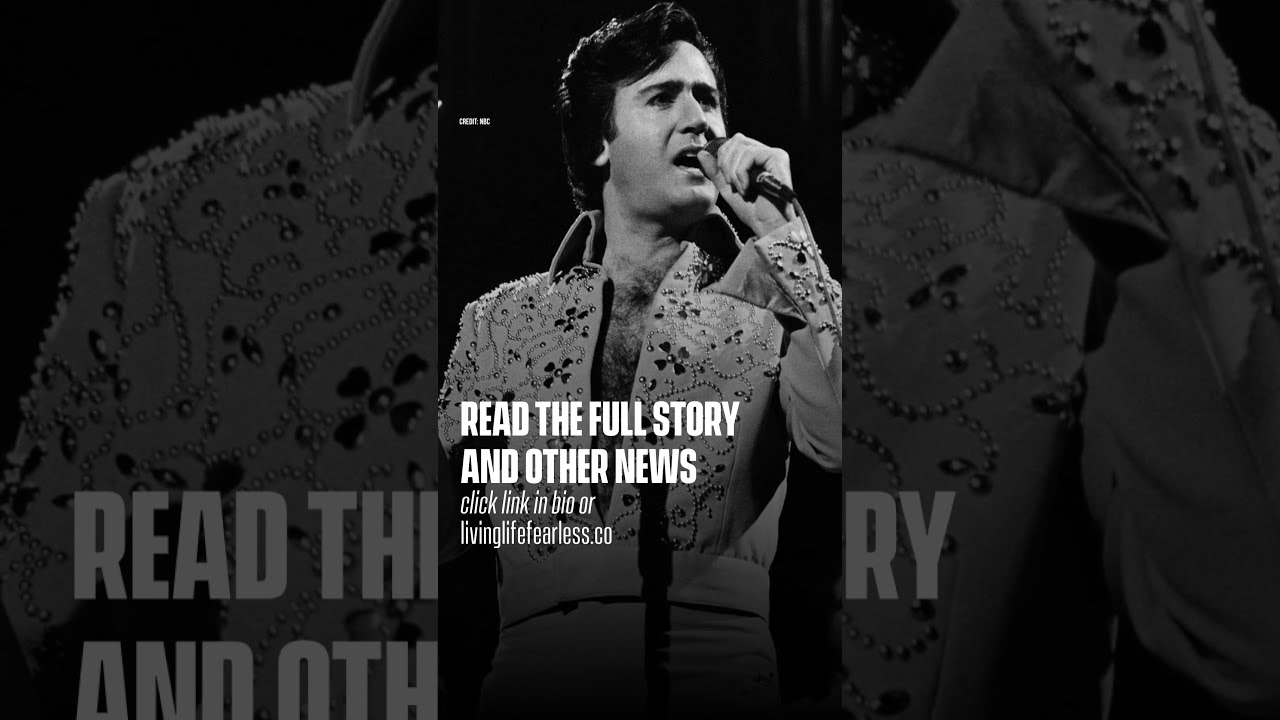In the black-and-white image, a man dressed in an elaborate, rhinestone-studded Elvis-style jumpsuit dominates the scene. Positioned centrally and taking up almost the entire photo, he is depicted from the waist up, gripping a microphone and appearing to sing passionately. His chest is exposed beneath the open suit, revealing chest hair, and his medium-length black hair is combed back. The background is entirely black, suggesting he might be on a stage. A blurred, cropped extension of his image frames the left and right sides, enhancing the focus on him. Text at the top left reads "credit NYC," and across the lower part of the image, it says, "read the full story and other news. Click link in bio or livinglifefearless.co," indicating the image may be a screenshot from a social media profile on a mobile device.